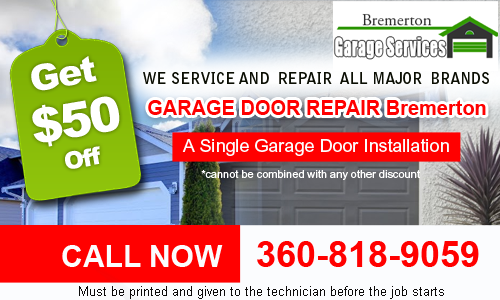Certainly! Here's a cleaned-up and detailed caption for the image:

---

The image depicts an advertisement for Bremerton Garage Services. Positioned at the top right, "Bremerton" is prominently displayed, with "Garage Services" just below it. The ad features a small illustration of the front of a house, highlighting a green garage door. On the left side of the image, there is a tag offering "$50 off." The promotion details include: "We service and repair all major brands of garage doors. Free $50 off single garage door installation. This offer cannot be combined with any other discounts." At the bottom of the advertisement, it instructs viewers to "Call now: 360-818-9059" and notes that the coupon "must be printed and given to the technician before the job starts."